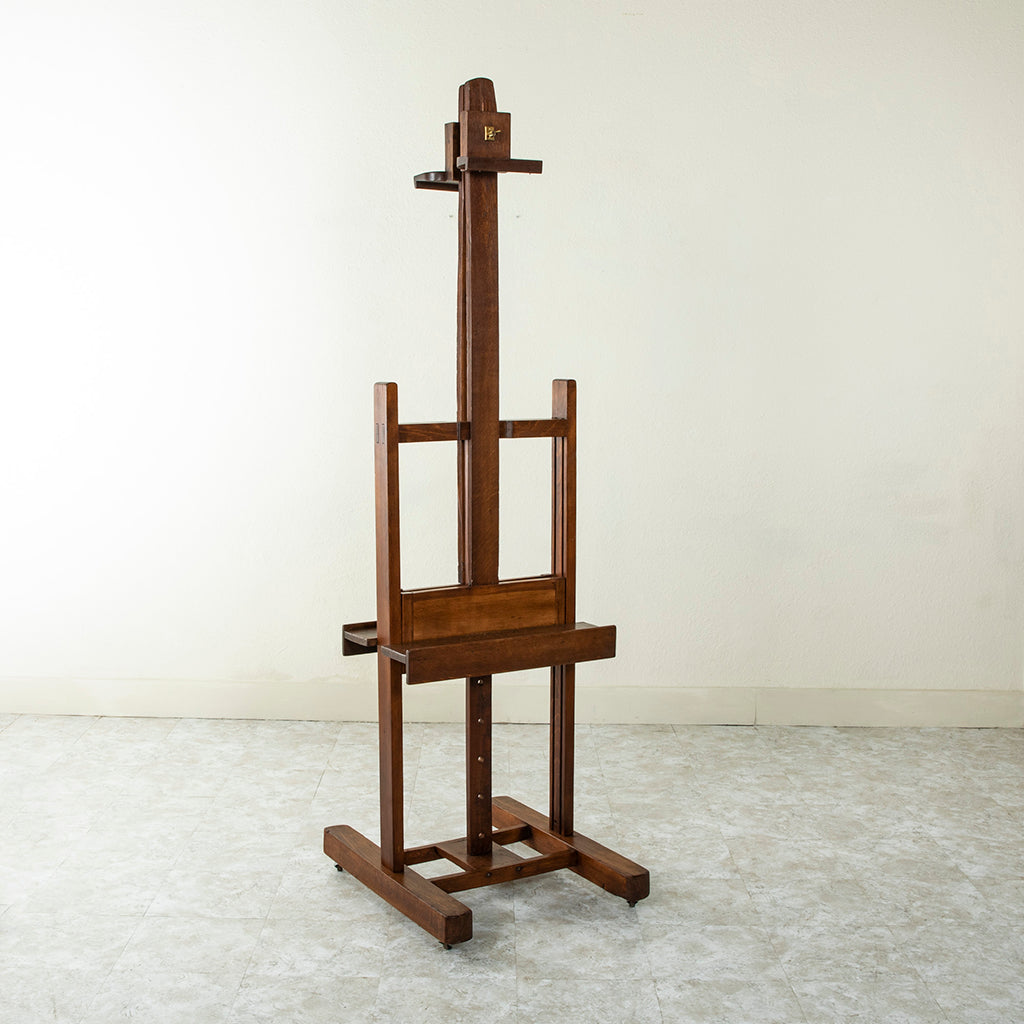The image depicts a tall, wooden artist's easel, prominently centered in a room. The easel, made of medium to dark brown wood, features a vertical support that extends upward to a clip designed for holding the top of a canvas. A horizontal ledge at the bottom serves as a base for the canvas and is likely adjustable to accommodate different canvas sizes. The base is structured in an 'H' design and there are additional vertical and horizontal supports for stability, some of which may include metal elements with holes, possibly for screws. It rests on a floor with light gray and mottled white or light brown tiles, suggesting a marble or slate texture. The background is a plain, cream or white wall with a gray baseboard at the bottom. There are no other objects in the room, emphasizing the easel as the central focus of the photograph. The entire setup casts a light shadow upon the floor, indicating a singular light source.